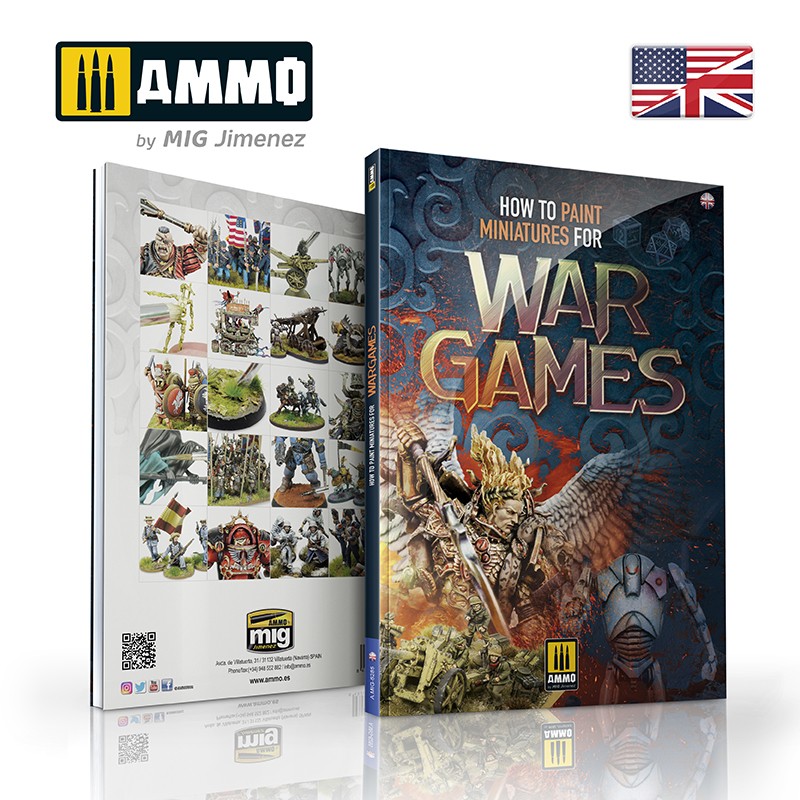This vertically rectangular, full-color image depicts the front and back covers of a book titled "How to Paint Miniatures for War Games." The background of the image is a plain white screen. In the upper left corner of the photo, there is a black and gold rectangle displaying the word "AMMO" in white with black bullets dotting the gold portion. The upper right corner features a split of the American and British flags.

The front cover of the book is notably detailed, with the title prominently displayed: "How to Paint Miniatures" in orange and "for War Games" in large, multicolored text occupying much of the cover. Surrounding the title are several vibrantly painted war game characters, some depicted as fantasy warriors with wings in yellow and red, and a metallic silver robot-like figure. 

The back cover of the book presents a collage of around 20 images illustrating the before-and-after transformations of the miniatures. The logo for "AMMO by Mig Jimenez" is present on both covers, emphasizing the brand. The books are situated on a reflective countertop, mirroring the covers on its surface.